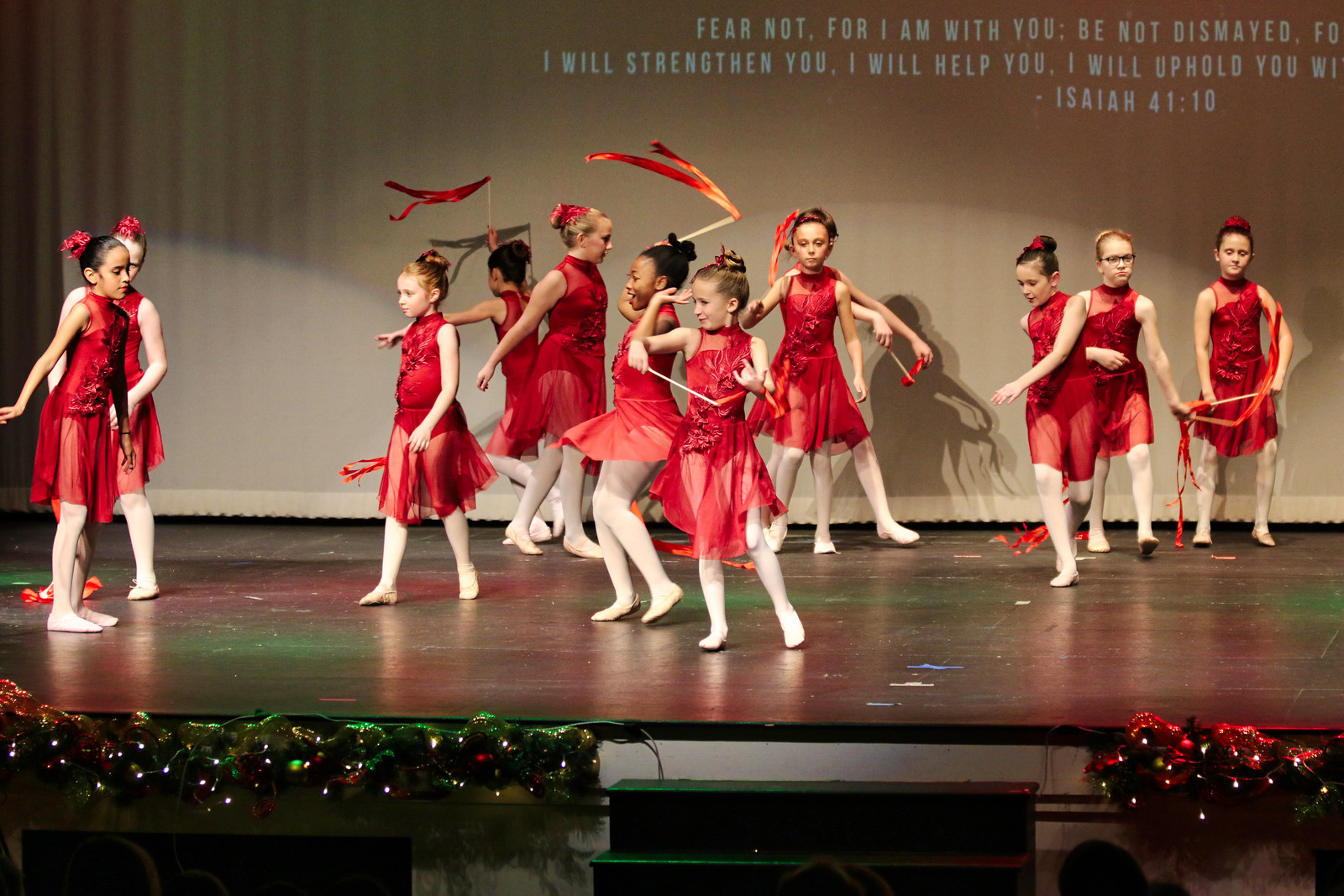The image is a horizontal rectangle depicting a school dance recital on a dark brown wooden stage. Eleven young girls with serious expressions are performing; they are wearing matching red dresses with white stockings, and most appear to be barefoot. Some hold thin metal batons, while others have small pairs of red flags. The stage is illuminated by stage lights casting red and green hues across the scene. In the background, against a light tan wall, a projected Bible verse from Isaiah 41:10 reads: "Fear not, for I am with you; be not dismayed, for I will strengthen you. I will help you. I will uphold you." Christmas garland with green foliage, red bows, and small white lights lines the front of the stage. Two dancers have collided on the right side, while two others stand close together on the left, with several more positioned centrally. There are stairs leading up to the stage on the side.